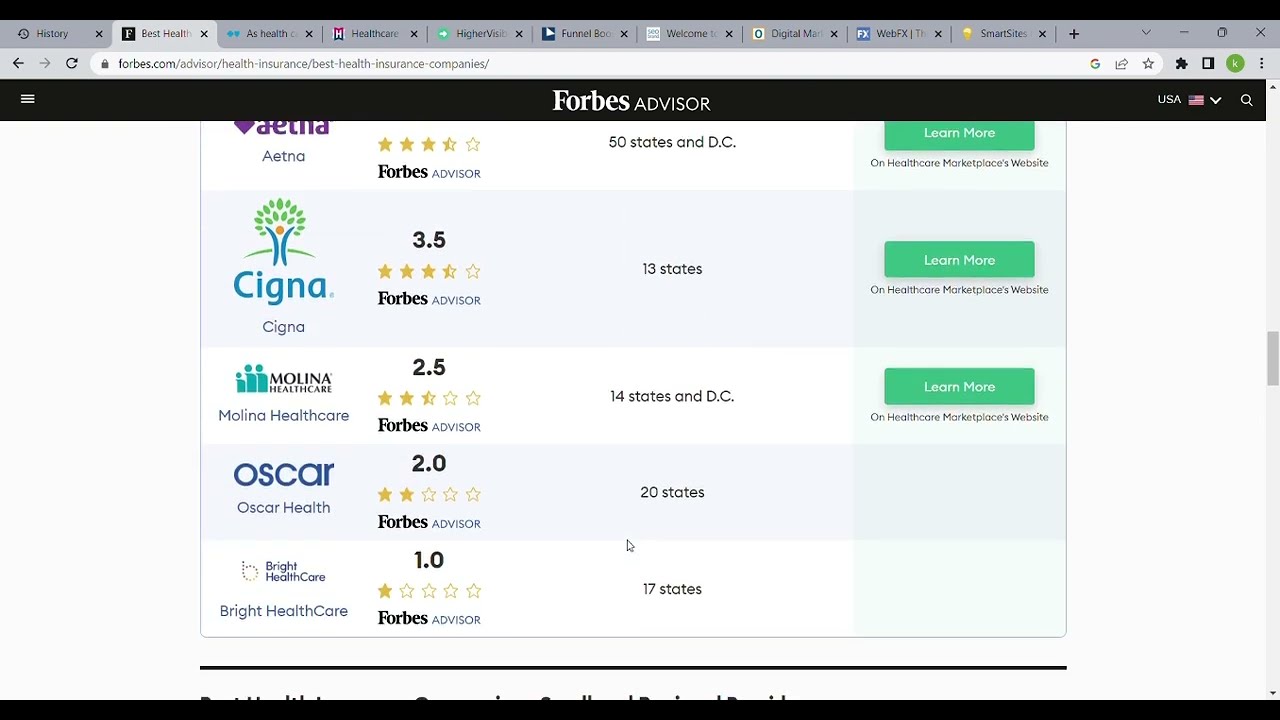This is a detailed screenshot from the Forbes Advisor website comparing health insurance companies. The screenshot, set against a white background, displays ratings for several healthcare providers. Each company is visually represented, with Aetna in purple, and Cigna, Molina Healthcare, Oscar Health, and Bright Healthcare in blue—all featuring their respective logos.

At the top, Aetna is shown with a 3.5-star rating and is available in all 50 states and D.C. Below Aetna is Cigna, also with a 3.5-star rating, covering 13 states. Molina Healthcare follows with a 2.5-star rating, available in 14 states and D.C., and Oscar Health with a 2-star rating, covering 20 states. Finally, Bright Healthcare receives a 1-star rating and is available in 17 states. Each company's section includes a green "Learn More" button for further information.

Above the main content, the webpage header reads "Forbes Advisor," and the URL visible in the address bar confirms it's from forbes.com/advisor/health-insurance-best-health-insurance-companies. There are multiple open tabs visible at the top of the browser. All the elements are centrally aligned on the page.